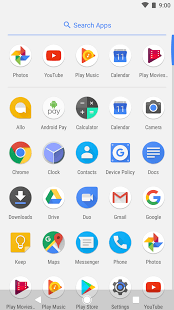This screenshot captures the search apps page on a cellphone, set against a light gray background. In the upper right corner of the image, there is a Wi-Fi signal icon, a battery indicator, and the time displayed as 9:00. The upper left corner is empty. 

Centered at the top, there is a blue magnifying glass icon beside blue text that reads "Search apps." Directly beneath this text, a thin blue line stretches horizontally across the screen. 

The app layout is organized into five columns and six rows. The first row features the following apps from left to right: a pinwheel icon, YouTube, an icon that might be for the phone app, Play Music, Calendar, and Play Movies. 

The subsequent rows list the following apps:

- Second row: Files, Android Pay, Calculator, Calendar, Camera, and Google Chrome.
- Third row: Clock, Contacts, Device Policy, Documents, Downloads, and Drive.
- Fourth row: Duo, Gmail, Google, Keep, Maps, and Messenger.
- Fifth row: Phone, Photos, Play Movies, Play Music, Play Store, and Settings.
- Sixth row: No apps listed in the provided description.

Overall, this screenshot provides a clear and organized view of the various applications available on the cellphone's search apps page.